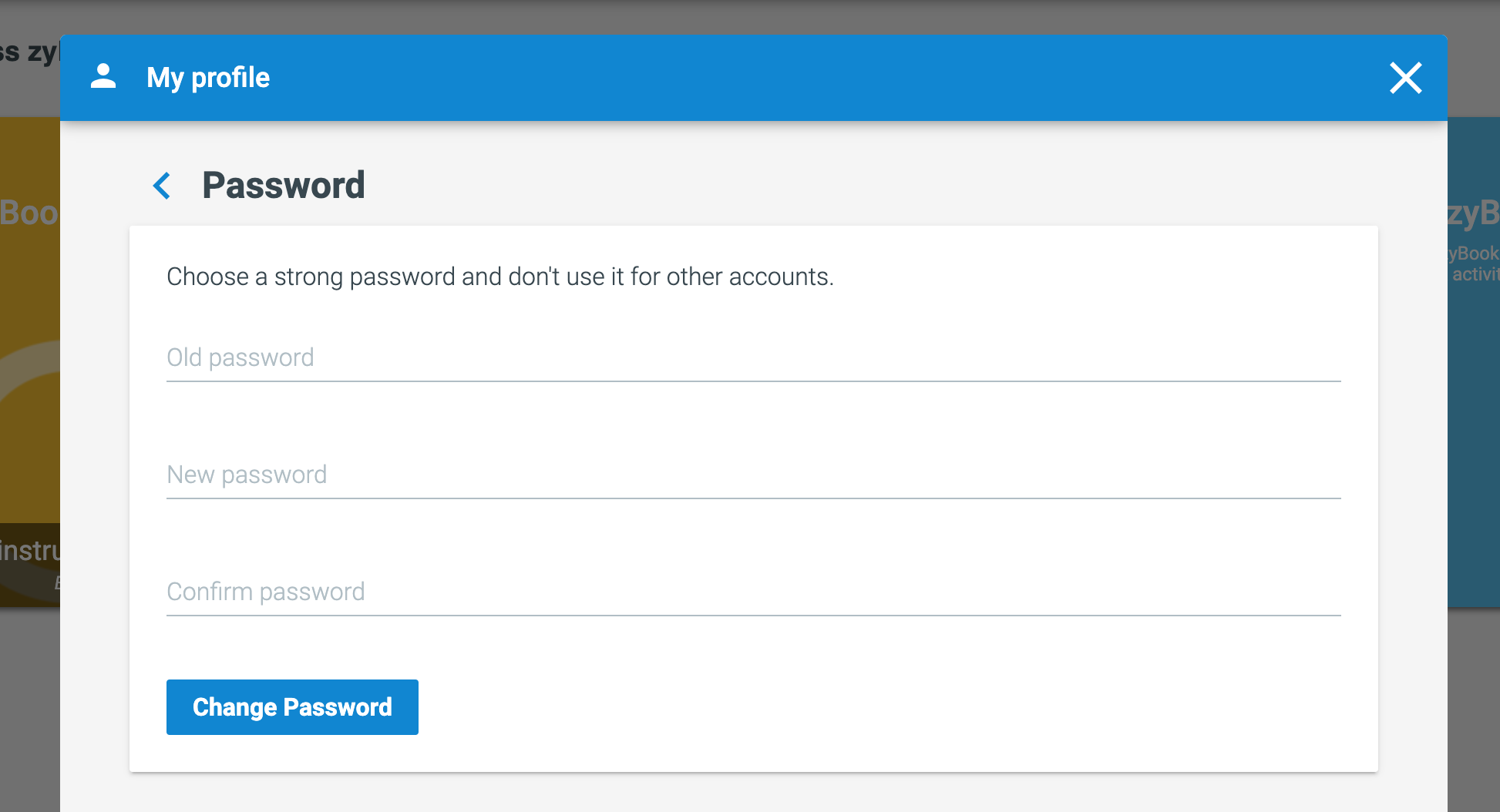This panoramic image showcases a password change interface. In the immediate foreground is a rectangular box with a long blue bar at the top. On this blue bar, a white circle with a half circle below it, representing a user profile icon, is prominently displayed. To the right of this icon, the white text reads "My Profile." At the far right end of the bar, a white "X" symbol is visible.

Beneath the blue bar, the background transitions to a grayish tone. Just below the bar, there is a black text label that says "Password." To the left of this label is a blue, sideways "V" symbol. Below the "Password" label, there is a white text box, outlined faintly in gray. Inside the text box, black letters instruct users to "Choose a strong password and don't use it for other accounts."

Further down, three sections are delineated by faint gray lines. The first section, labeled "Old Password," is followed by a gray input line. Next is the "New Password" section, also accompanied by a long gray input line. Lastly, the "Confirm Password" section has another long gray input line for re-entering the new password.

At the bottom left of this interface is a blue rectangular button with the white text "Change Password." The background of the image reveals a partially visible, grayed-out webpage, indicating that this password change popup is currently active, preventing any interaction with the underlying page content.

Overall, this image clearly depicts a webpage where a user can change their password, with detailed instructions and input fields provided for the old, new, and confirm password entries.